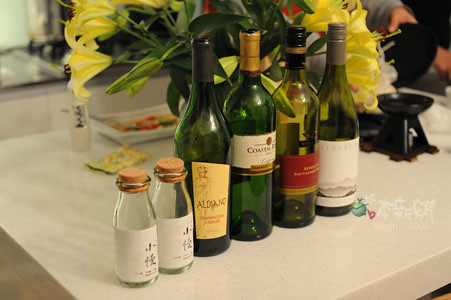This is a detailed photograph of a dinner table covered with a white tablecloth, viewed from a slight angle above. In the foreground, a lineup of various bottles is prominently displayed. On the left, there are two short, old-fashioned milk jug-shaped bottles with brown tops and white labels featuring Japanese text. Following these are four different green wine bottles, each with distinct characteristics: the first tall green bottle has black foil around the top and a label that seems to read "al denno," the second has gold foil, while the third and fourth lighter green bottles have black and gray foil respectively, with one featuring a red label and a larger white label.

Behind this array of bottles sits a bouquet of yellow lilies, adding a splash of color to the scene. To the upper right of the flowers, you can glimpse a small black chafing plate with a candle underneath, presumably for warming food. Adjacent to the flowers, on the left side, is a rectangular white appetizer plate containing various colorful foods. The top right corner of the image captures a partial view of a person's hand holding a round black plate. The image also contains an intricate watermark in Japanese, incorporating a small logo resembling a traditional sake bottle and a red icon, albeit faint against the white tablecloth.